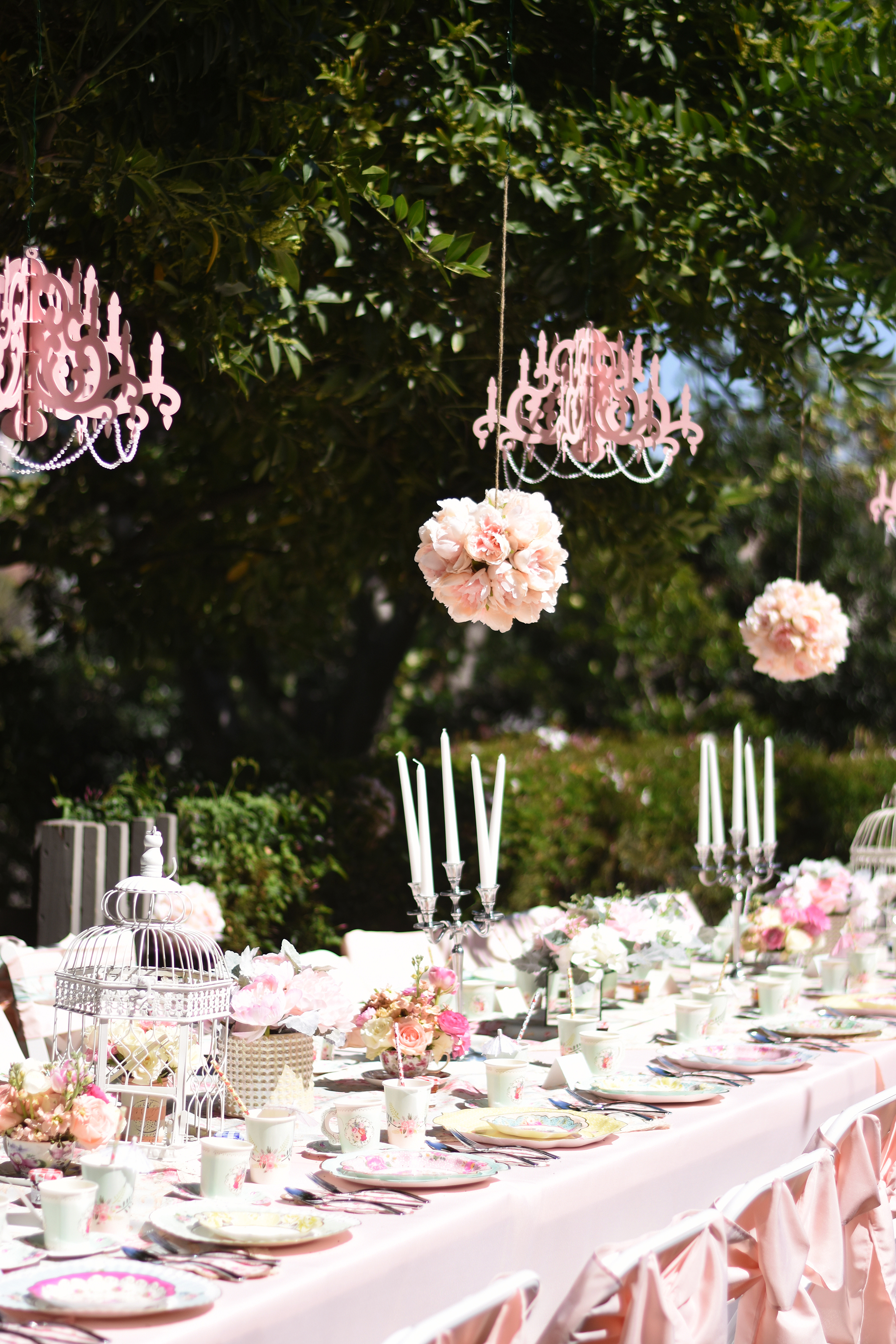The photograph captures an elaborate outdoor table set for a garden event, possibly a wedding. The table is long and adorned with a pink tablecloth, set with ceramic plates, cutlery, floral printed paper cups, and small cups with paper straws. Each wooden folding chair is decorated with a pink covering and a bow on the back. The centerpiece of the table features silver candelabras holding tall white candles, interspersed with short vases of pink and white roses. 

Suspended above the table from the branches of an overhanging tree are whimsical pink cardboard chandeliers, one in the upper left, another just right of the center, and a blurry one further in the background. Flowers, shaped into balls and resembling large hanging bouquets of carnations or roses, are also suspended from the tree, creating a magical canopy effect. Additional decor includes fake birdcages and floral vases along the length of the table. Overall, the entire scene is set against a backdrop of lush green trees and a hedge, bathed in the sunlight of a clear day, conveying a festive, sophisticated ambiance.